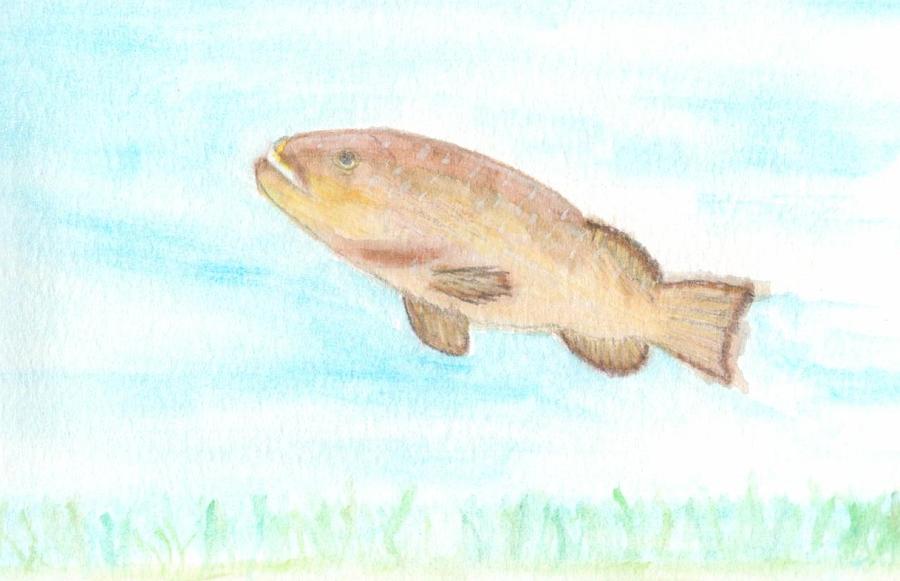The image is a detailed pencil and crayon drawing of a fish underwater. The fish, primarily light and dark brown with hints of yellow around its mouth, is angled as if swimming upwards, with its left side higher than its right. The fish has a single, visible black eye and an open mouth, revealing part of its front fin and tail. The background is a blue-white hue representing water, with blue and green seaweed or sea grass growing underneath the fish. The fins, tipped in dark brown, and the grass add a vibrant, natural touch to the underwater scene. There are no words or numbers in the image, and it is brightly lit, making all details clear and vivid.